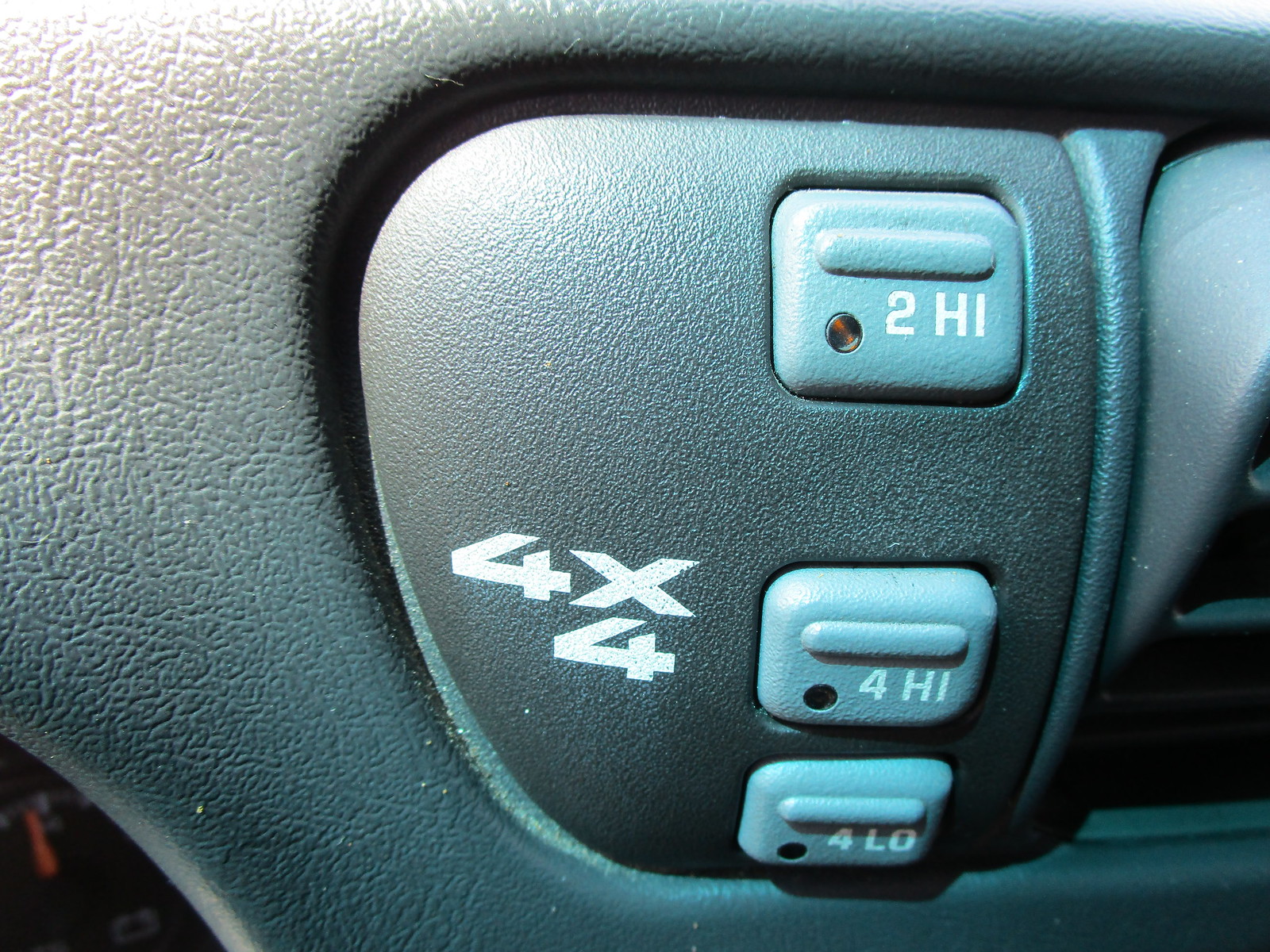This up-close photograph captures a section of a vehicle's dashboard, characterized by a dark bluish-gray textured surface. Prominently displayed in white lettering are the numbers and letters "4X4," possibly highlighting the vehicle's four-wheel-drive capability. Central to the image are three small, squarish buttons, each a light blue-gray color with a small reddish circle, presumably indicative of lights that are currently not illuminated. The top button bears the label "2 HI," while the two buttons positioned beneath it are labeled "4 HI" and "4 LO" respectively. Additionally, partially visible on the right side of the photograph is an air vent, suggesting this section lies within a functional and possibly dusty vehicle interior.